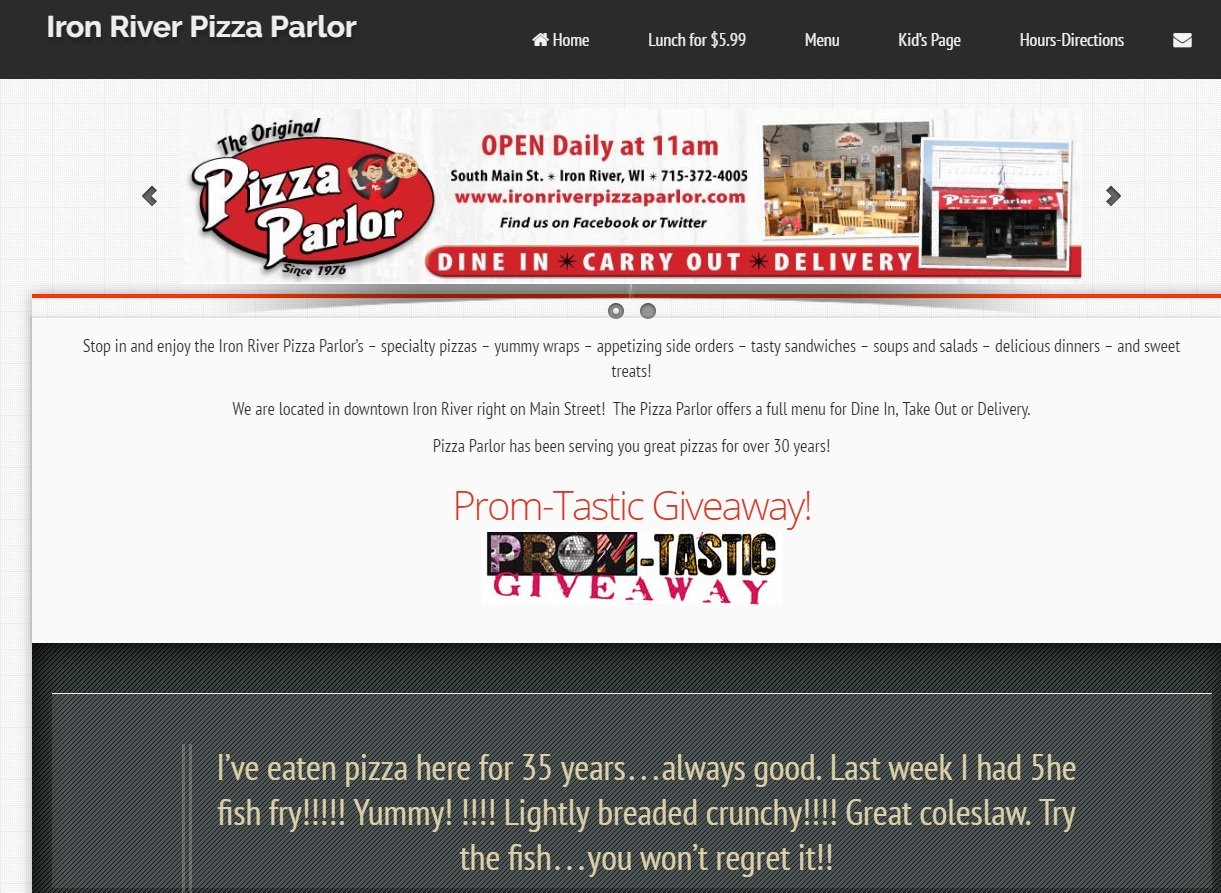Screenshot of the Iron River Pizza Parlor Website

In this detailed screenshot of the Iron River Pizza Parlor website, the layout is efficiently designed to guide users through the various sections. At the top left, the title of the website, "Iron River Pizza Parlor," is prominently displayed. 

To the top right, a navigational bar features multiple tabs arranged from left to right:
- "Home"
- "Lunch for $5.99"
- "Menu"
- "Kids Page"
- "Hours & Directions"

Adjacent to these tabs is an envelope icon, likely a link for users to send emails directly to the pizza parlor.

The upper part of the webpage showcases the brand's logo on the left, with "Pizza Parlor" written in giant white text. Above this text is the phrase "The Original Pizza Parlor," emphasizing its authenticity, and below it, the tagline reads "Since 1976," highlighting the establishment's long-standing presence.

The logo is adorned with a cheerful character—a man in a red cap and shirt who is holding up a pepperoni pizza in his left hand—capturing the essence of the pizzeria. Centrally located on the page is an announcement stating, "Open Daily at 11 AM," ensuring customers are aware of the opening hours. Below this, the address is provided: South Main Street, Iron River, Wisconsin, along with a phone number for inquiries: 715-372-4005. At the very bottom, there is a direct link to the website for easy access.